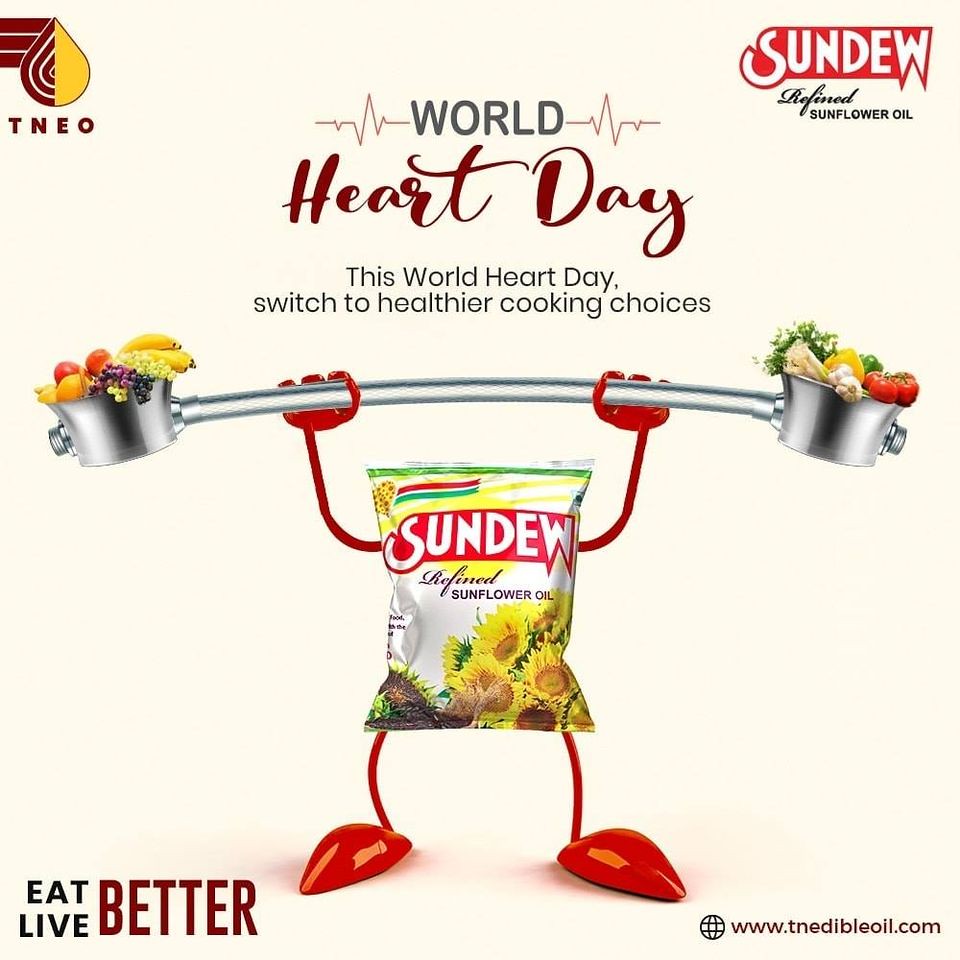The image features an advertisement for Sun Dew refined sunflower oil against a very light pink background. The centerpiece of the ad is the sunflower oil package, designed with playful illustrations of red arms and red legs, mimicking a person holding up weighted bowls on each side of a silver metal bar. These bowls contain a variety of fruits and vegetables, including yellow bananas, yellow lemons, purple grapes, red tomatoes, and other green items, emphasizing healthy choices.

The package itself is predominantly white, with striking red, yellow, and green accents. The front of the package displays the Sun Dew brand name in white letters on a red background. Below this, "refined sunflower oil" is printed in black letters. A small black and yellow symbol marked "T-N-E-O" is positioned on the left side of the package. The top of the ad features the message "World Heart Day" in gray letters, followed by the tagline "Switch to healthier cooking choices" in black.

At the bottom left corner of the package, the phrase "Eat, Live Better" is printed in black letters, promoting the health benefits of the product. The website www.tnedibleoil.com is listed in black on the bottom right corner, directing viewers to more information. The overall white background and colorful design elements create an eye-catching and informative ad encouraging healthier dietary choices in honor of World Heart Day.